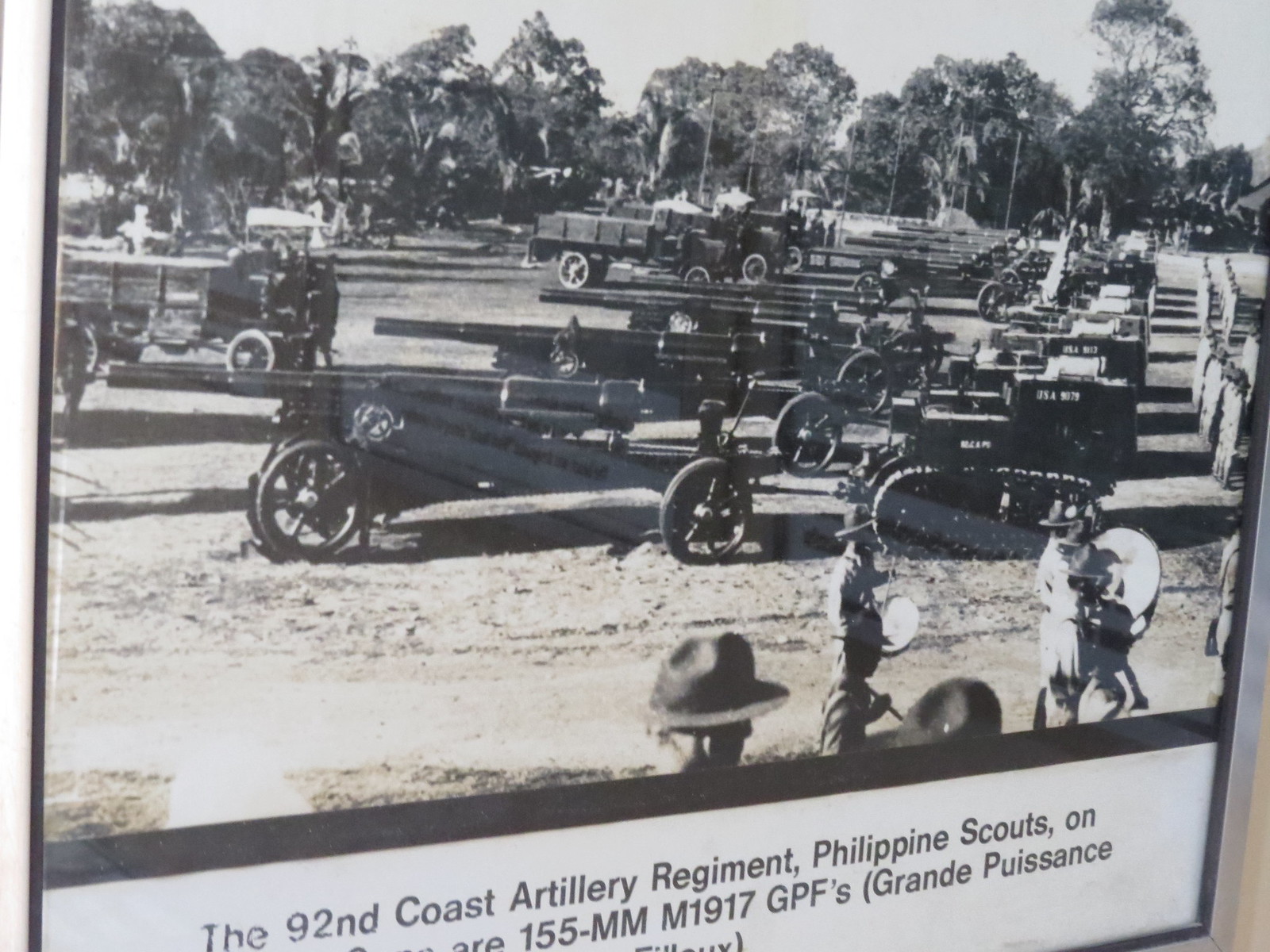This detailed black-and-white photograph, encased in a silver frame with glass that reflects light, shows a wartime scene preserved on what seems to be a cream or off-white wall. In the foreground, there is a large, open dirt field lined with several imposing cannons and smaller tanks, their barrels not raised. To the left, an old military truck with thin tires contrasts with the distant military cars and trucks scattered further back. At the top center of the image stands two more cannons, amidst tall, leafy trees, suggesting a summertime setting. On the lower right of the frame, a group of marines or soldiers in uniformed ranks wear distinctive cowboy-like hats and stand next to marching drums, collectively looking to the right. Below the image, a white rectangular caption reads in stark black text: "The 92nd Coast Artillery Regiment, Philippine Scouts," followed by partially obstructed and cut-off letters, indicating "155-mm M1917 GPF (Grande Puissance)."